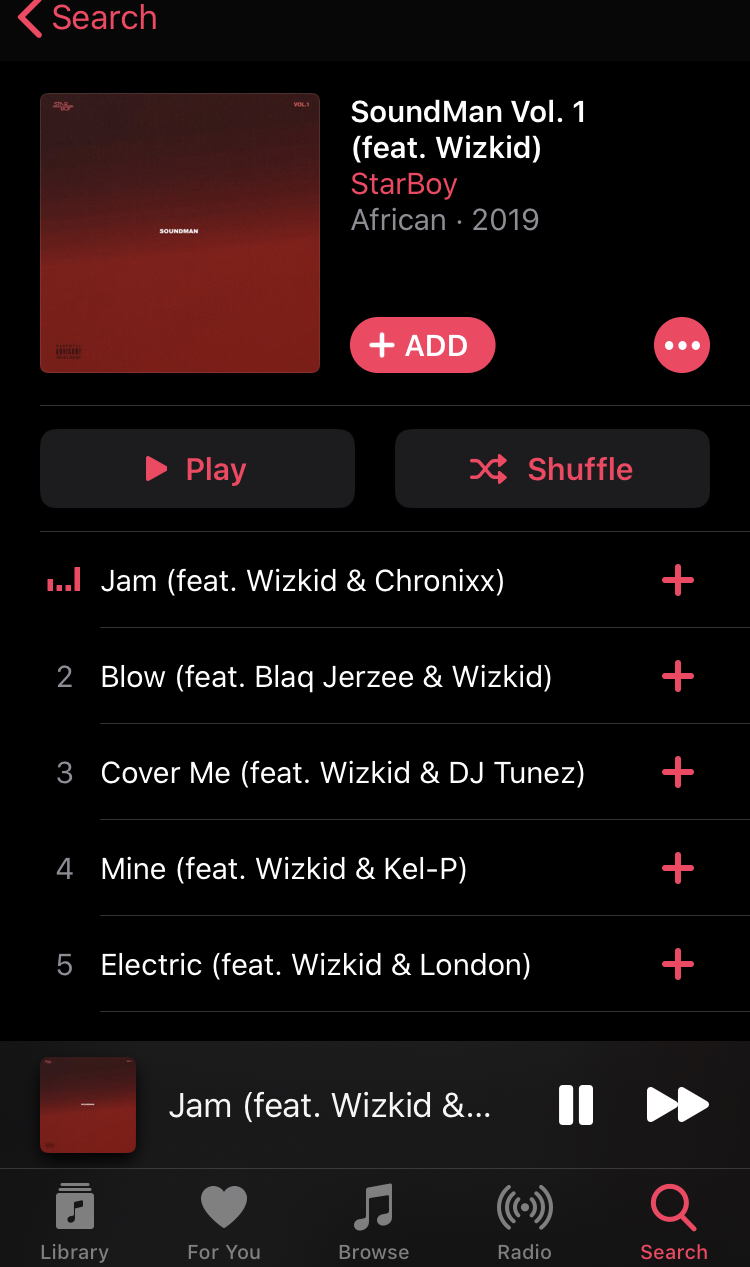This image is a screenshot of a music application displayed on a phone. The top left corner of the screen features a section with a black background, showcasing a pink arrow pointing to the left. Beside this arrow, in pink text, is the word "Search." Below this, on the left half of the screen, is an album cover that is square-shaped with rounded corners. The album cover has a red gradient background, transitioning from brighter red at the bottom to darker red at the top. Centered within the cover is a small piece of white text reading "Soundman." Additionally, there are pink text elements located in the top left and right corners, and black text in the bottom left corner of the album cover.

To the right of the album cover, white text indicates "Soundman Vol. 1" (with "Vol." abbreviated). Beneath this title, in parentheses, the text "(feat. Wizkid)" is displayed. Further below, pink text reads "Starboy," followed by gray text that provides the genre "African," a gray dot, and the release year "2019."

Aligned with the bottom edge of the album cover, a pink pill-shaped button on the left side of the screen contains white text that says "ADD" in capital letters, accompanied by a white plus sign to its left. On the right side of the screen, at the same level, there is a round pink button featuring three white dots arranged horizontally.

Below these buttons, a medium gray separator line spans the width of the screen. Continuing downward, there are two light gray rectangular buttons with rounded corners, both containing pink icons and text. The button on the left reads "Play" and includes a pink triangle icon indicating play. The button on the right reads "Shuffle" and includes a pink shuffle icon composed of two arrows twisting across each other, pointing to the right.

A second separator line appears beneath these buttons, and below it, the tracks are listed out, continuing the detailed layout of the application interface.